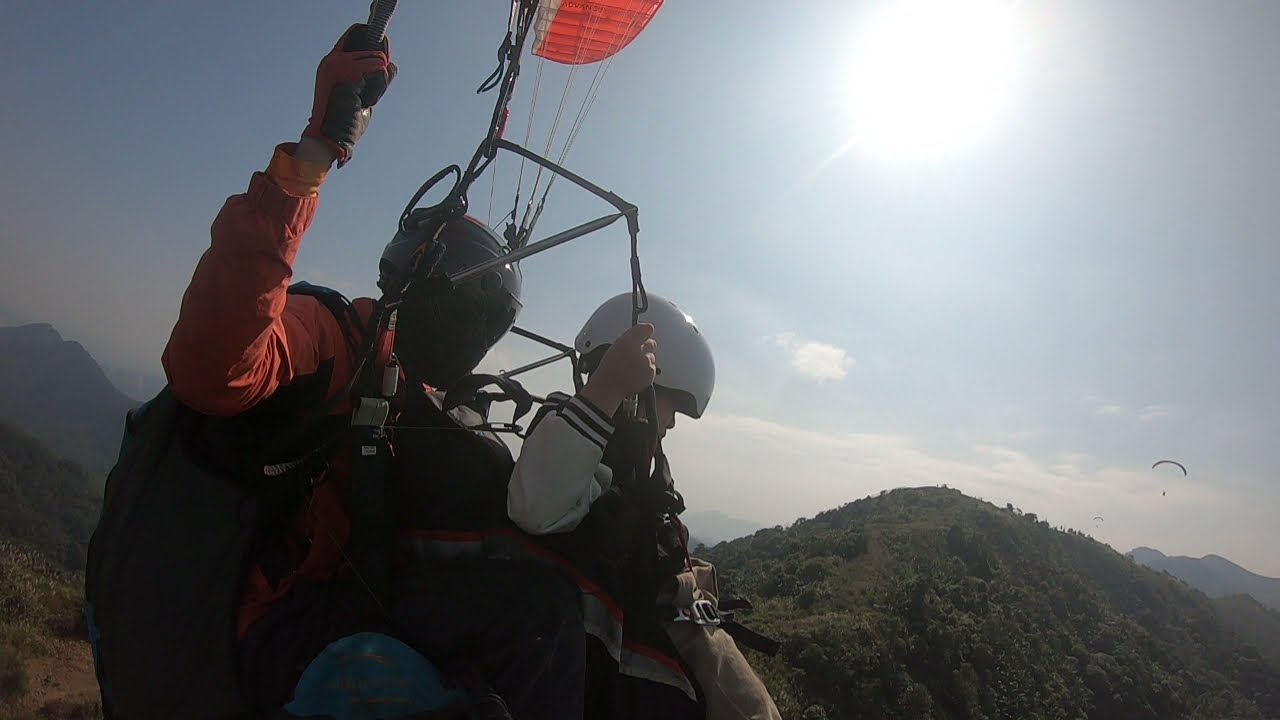The picture captures a bright and sunny day, showcasing a man and a child engaged in the thrilling activity of hang gliding. They are suspended in mid-air with a distinct orange and white parachute billowing above them. The man, positioned at the back, is clad in an orange coat and a black helmet, while the child, sitting in front, dons a green and white coat paired with a white helmet. Both are securely strapped in, ensuring their safety as they glide gracefully. The backdrop features picturesque rolling hills adorned with trees and bushes, interspersed with patches of bare dirt. Off in the distance, another parachute is visible, highlighting other adventurers in the sky. The scene is bathed in the bright sunlight, which casts a hazy glow over the landscape, adding to the serene and exhilarating atmosphere.